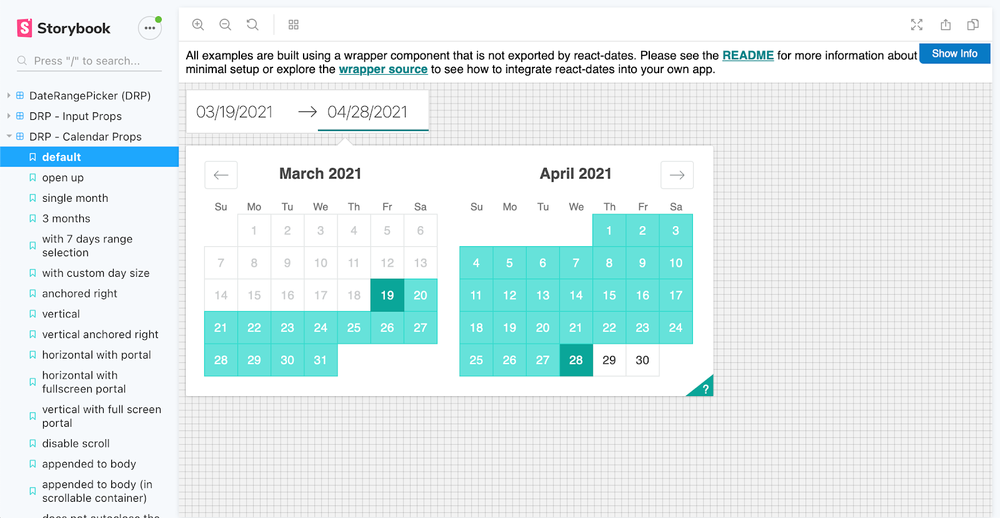In the image, the top left corner prominently displays the website's name, "Storybook". To the left of the name, there's a small rectangular icon with a pink background featuring an 'S'. Adjacent to the icon is a circular button with three vertical dots; a smaller green circle overlays the top right of this button. Beneath this, a search bar invites the user to "Press F to search...".

The interface below is divided into three main categories. The first category is labeled "Date Range Picker, DRP", followed by "DRP Input Props", and lastly "DRP Calendar Props". Under the "DRP Calendar Props" section, numerous subcategories are listed: "Defaults", "Open Up", "Single Month", "Three Months", "With 7 Day Range Selection", "With Custom Day Range", "Anchored Right", "Vertical", "Vertical Right", "Horizontal with Portal", "Horizontal with Fullscreen Portal", "Vertical with Fullscreen Portal", "Disable Scroll", and "Appended to Body".

The central area of the page features two side-by-side calendars, March 2021 on the left and April 2021 on the right. The current date, March 19th, is highlighted on the March calendar, while the April calendar has the 28th highlighted.